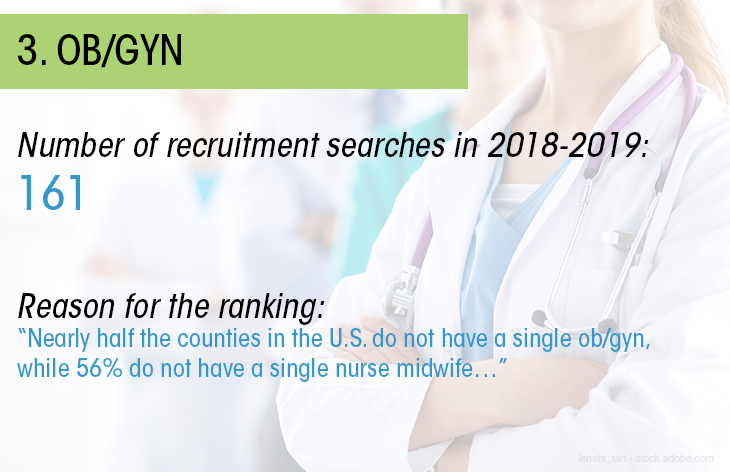The image is an informational slide highlighting statistics related to OBGYN recruitment and availability in the U.S. In the background, there is a semi-faded stock photo of a female doctor or nurse, dressed in light blue scrubs, a white lab coat, and a stethoscope around her neck. She stands with her arms crossed and is primarily visible from the neck down, with her hair pulled back in a ponytail. A green text box at the top left reads "3.0B.GYN," followed by a caption in black text stating "Number of recruitment searches in 2018-2019: 161," with the number "161" in blue. Below this, another caption explains the "Reason for the ranking:" with the text in blue detailing that "nearly half of the counties in the U.S. do not have a single OB-GYN, while 56% do not have a single nurse midwife." This information is intended to showcase OB-GYN and nurse midwife statistics, emphasizing the shortage in many U.S. counties.